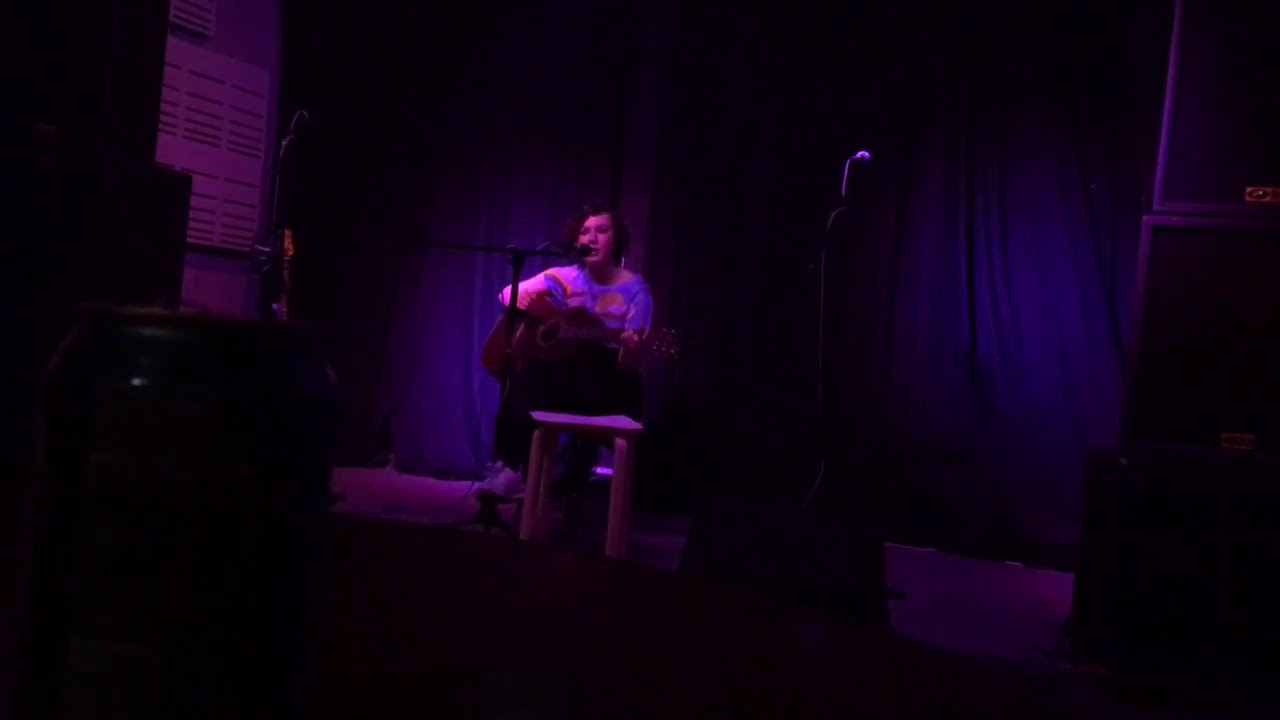The image captures the dimly-lit atmosphere of a one-woman concert, emphasizing the deep purplish-pink tones that drench most of the scene. At the center of the stage sits a young lady with short hair just above her chin, playing an acoustic guitar. She is wearing a light-colored shirt adorned with a rainbow and sun design, paired with dark pants and white sneakers. The backdrop features a blue draped curtain and a board with lines, barely visible in the dim lighting. Positioned in front of her is a microphone stand at which she sings, her mouth open and engaged with the audience. To her left are additional speakers and an unused microphone, while a small wooden stool or table stands before her, seemingly without purpose. The photographer's perspective, taken from the audience, captures the essence of an intimate performance set against a backdrop of shadows and colored lights.